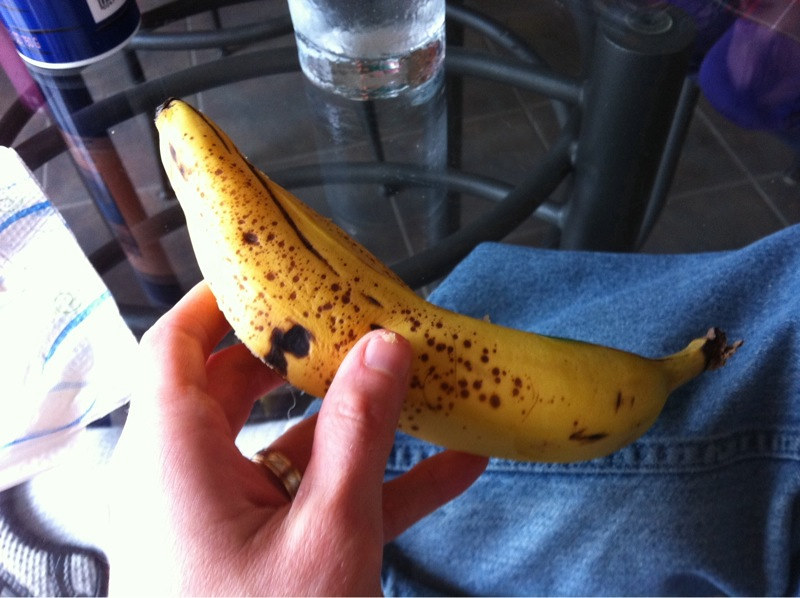In this image, a person is holding a very ripened banana. The banana has a multitude of brown spots, indicating it is overly ripe, with a particularly dark, almost black bruised area between the thumb and fingers. The stem end of the banana points downward towards the person’s leg, which is clad in horizontal blue jean seams suggesting a relaxed, cross-legged sitting position, possibly with one leg propped up.

The person’s thumb is visible on top of the banana, while their four other fingers support it from underneath. The hand in focus wears a silver or platinum-colored wedding ring on the fourth finger, notable for its intricate edging.

The person appears to be seated at a glass-topped table with a black metal frame. On the table, there is a glass of clear liquid with condensation, implying that the liquid is cold. Next to the glass, part of a dark blue can is visible, though its label is indistinguishable. Near the person’s hand, there is a paper towel or some paper-textured item at the table’s edge.

In the top right corner of the image, a few blurry items are scattered on the floor, which is covered in dark gray or possibly black tiles with a design of small squares. The overall setting suggests an informal, comfortable environment where the person is casually examining the overly ripened fruit.